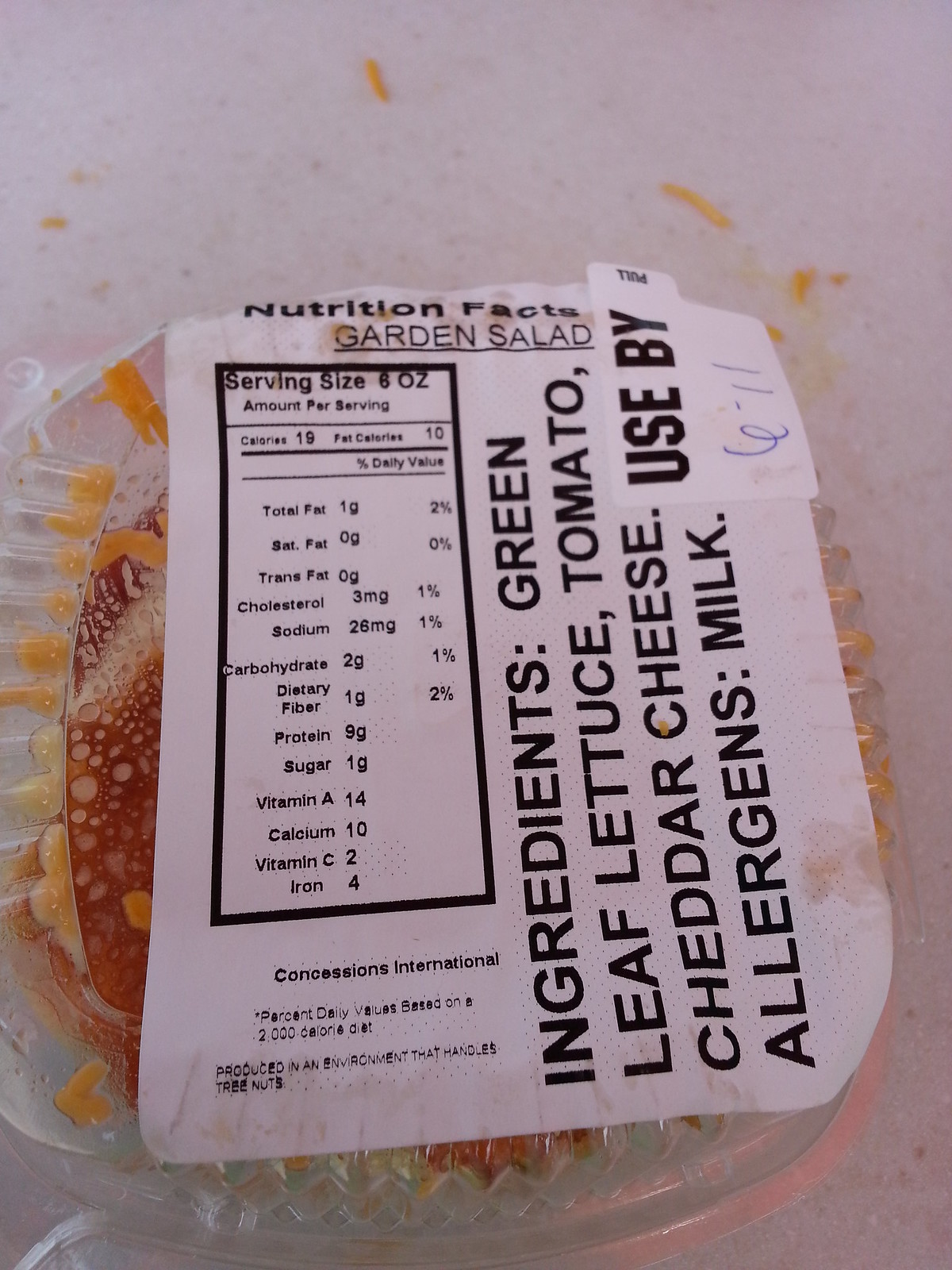Close-up of a garden salad container with visible nutrition facts on the label. The serving size is 6 ounces, containing 19 calories and 10 from fat. The salad has 1 gram of total fat, including no saturated or trans fat, 3 milligrams of cholesterol, and 26 milligrams of sodium. It provides 2 grams of carbohydrates, 1 gram of dietary fiber, 9 grams of protein, and 1 gram of sugar. Nutrient content includes 14 grams of Vitamin A, 10 grams of calcium, 2 grams of Vitamin C, and 4 grams of iron. The salad consists of green leaf lettuce, tomato, and cheddar cheese, with milk listed as an allergen.